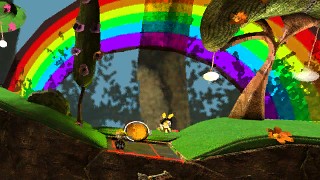This is a vivid, cartoonish landscape drawing that features a small road cutting through two lush green hills. On the left hill stands a tall tree adorned with tiny pink flowers and accompanied by a bush. The right hill hosts a larger tree with a wider trunk and a broad canopy. The backdrop is dominated by a dark sky, from which a large, brilliant rainbow arches, displaying the full spectrum of colors: red, orange, yellow, green, blue, and violet. This rainbow stretches from the back of the left hill to the back of the right hill, creating a diorama-like scene. In the center of the picture, behind the horizon, is a large tree stump, with silhouettes of leaves scattered in the background. The ground appears to be cut away, revealing the soil beneath the hills. The overall image has a whimsical and detailed cartoon aesthetic.